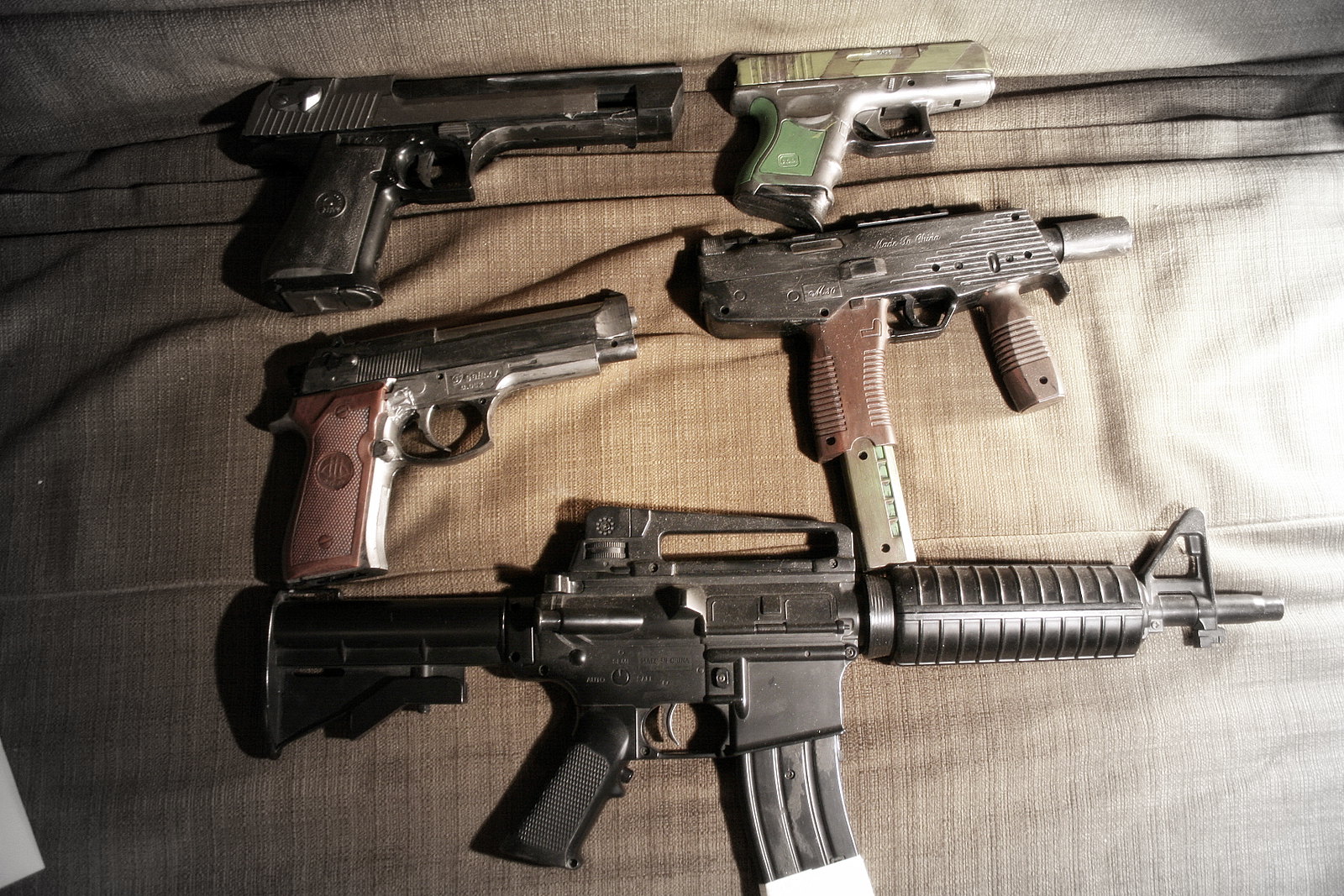This color photograph depicts a collection of five firearms laying on a dark brown or grayish cloth, potentially a couch cushion. At the bottom of the image is a miniaturized M16 type assault rifle with a noticeably short barrel, facing right. It has a magazine inserted and is in a dark grayish color. Positioned above and to the right of this M16 is a MAC-10 machine gun, distinguished by its stainless steel extended magazine and brown handle and forward grip. Nearby, there are three semi-automatic pistols: one directly to the left of the MAC-10, featuring a black slide and brown grip; a small concealed carry pistol with yellow and brown camouflage striations and a green grip, situated in the top right; and another dark gray larger pistol. This varied collection of guns, including both semi-automatic and single shot models, is displayed on a fabric background, creating a striking and detailed still life of weaponry.